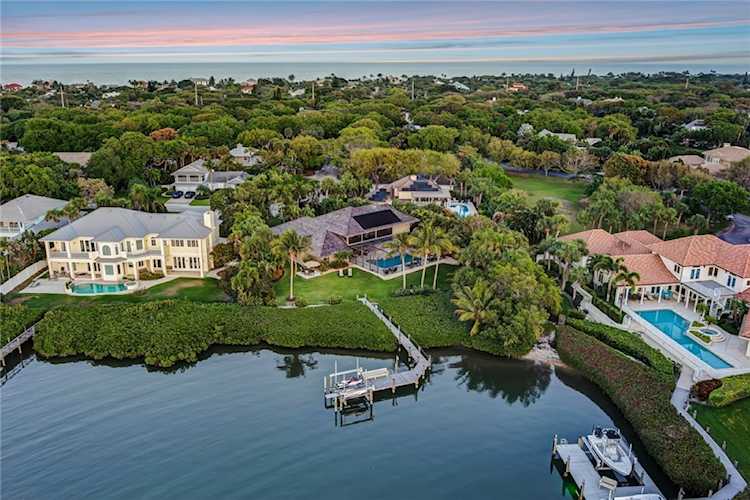This aerial photograph captures an opulent tropical resort area, featuring an array of multi-million dollar mansions nestled amidst lush greenery. The estates, characterized by their expansive multi-story structures, luxurious gardens, and private swimming pools, stretch across a scenic inlet. Each mansion boasts its own dock, accessible via both cement and wooden walkways, with some docks even blending seamlessly into the landscape due to high-grown bushes. At the forefront of the image lies a serene body of water with gentle ripples, while the upper section reveals a distant view of the sea meeting the sky. Notable details include a two-story house on the far left with a grassy walkway to its pier, a house on the right adorned with a red tile roof and an adjacent speedboat, and another central mansion framed by majestic palm trees. The meticulous arrangement of private jetties and the presence of multiple pools underscore the affluence of this picturesque neighborhood.